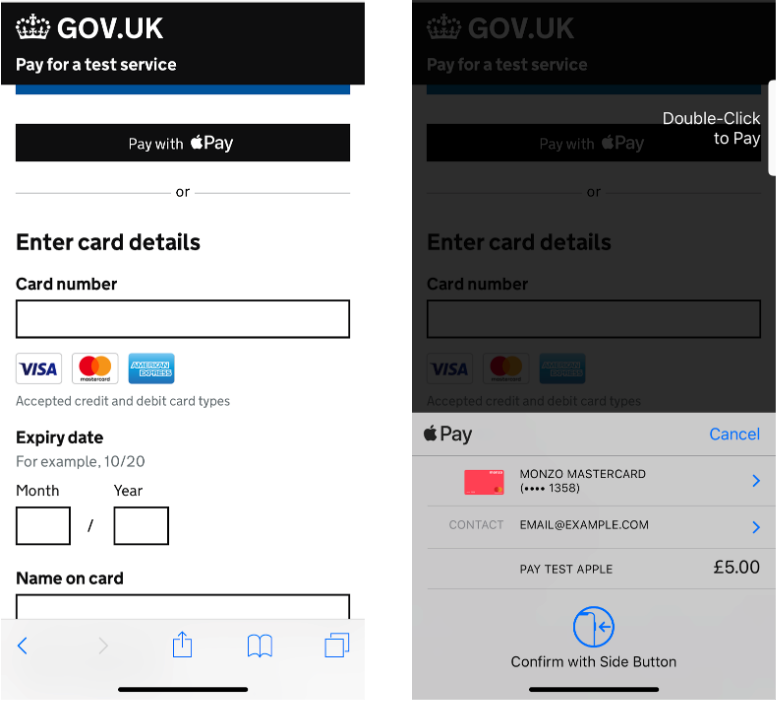The image is a composite of two screenshots taken from a mobile phone in portrait mode, presenting a step-by-step process on a payment page from the gov.uk website.

**Left Screenshot:**
- Across the top, a black banner with white text reads "gov.uk" with a crown symbol, followed by "pay for a test service."
- Directly below, a thin blue banner spans almost the entire width, though it contains no text.
- A larger black banner beneath displays "Pay with Apple Pay," accompanied by the Apple logo.
- The middle of the screen features a grey line followed by "or" and another grey line, all in grey.
- Below this, the section to manually enter card details starts with fields for "card number" and provides a long, oblong box to fill in the card number.
- Acceptable card types, Visa, MasterCard, and American Express, are indicated with their respective logos, accompanied by the text "accepted credit and debit card types" in grey.
- Further down, in bold black text, "expiry date" is specified, with an example format "10/20" in grey, and input fields labeled "month/year."
- The next section requires "name on card" with another oblong box for input, though partially obscured by the screen edge.
- At the bottom are standard mobile navigation icons: a blue back arrow, a greyed-out forward arrow, a share/upload icon, a blue book icon, and a multi-square file icon.
- A thin black line is centered at the bottom.

**Right Screenshot:**
- The right portion shows progression in the payment process, retaining the same background elements with a slight dark overlay, indicating a step forward.
- The top still displays "gov.uk" and "pay for a test service" followed by "pay with Apple Pay" and the alternate option to "enter card details."
- Overlaying the darker background, halfway down on the left, is the Apple logo with "pay," and on the right, "cancel" in blue text.
- Below, there's an icon of a Monzo MasterCard in red, labeled "Monzo MasterCard."
- Additional details include an obscured card number, displayed as "****1358," with a blue arrow pointing right.
- Contact information is specified as "email@example.com," with another blue arrow.
- The payment section shows "pay test Apple" and "£5" on the right side.
- Instructions at the bottom prompt "confirm with side button," illustrated with an icon depicting the right side of a mobile phone and an arrow pointing to its side button.
- Overlaying this area is the instruction "double-click to pay."

In summary, the composite image depicts a detailed step-by-step process for paying through Apple Pay on a gov.uk page, transitioning from card details entry to double-click confirmation with Apple Pay.